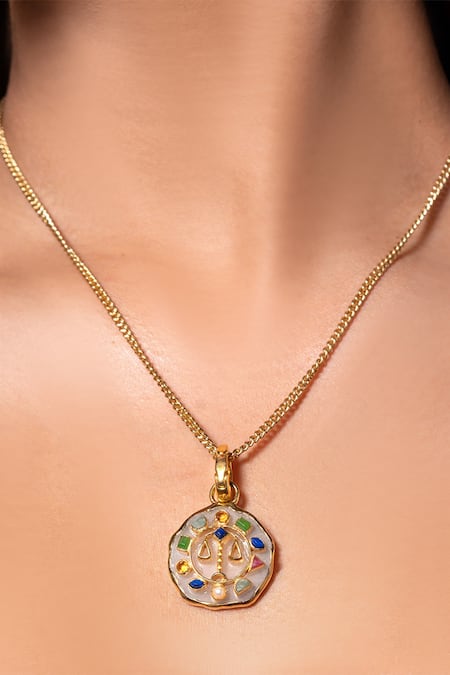This close-up image features the neck and upper chest area of a young, white woman, showcasing a unique necklace as the primary focus. The necklace consists of a thin gold chain with a gold clasp attaching a distinctive medallion. The pendant is a gold circle with a slightly jagged edge, giving it a handmade, almost primal appearance. At its center, there is an intricate design of old-fashioned scales, symbolizing balance, created with gold wiring. Encircling the scales is a blue diamond shape set against a white circular background, resembling sea glass.

Surrounding this central design are a series of different colored gemstones arranged in a pattern reminiscent of clock numerals. Starting at the top and moving clockwise, the gems include a yellow jewel, followed by green, blue, pink, light bluish gray, a pearl at the bottom, another blue, yellow, green, and finally that same grayish blue shade. The thoughtful arrangement and variety of colors add to the medallion's unique and captivating appearance.